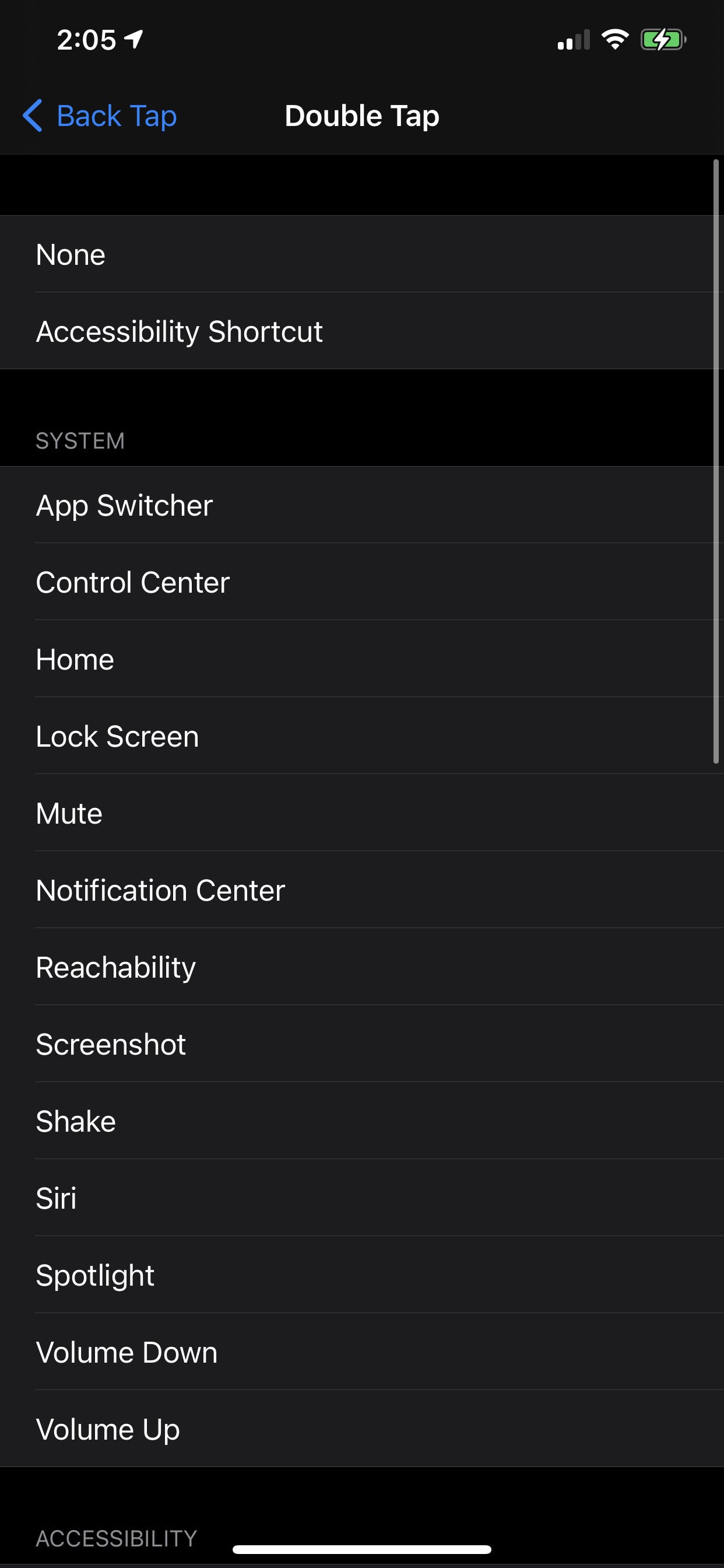The image is a screenshot taken from a mobile phone screen, displayed at 2:05 PM with a full battery charge. At the top of the screen, the text "Double Tap" is visible, followed by options indicating "None" for the accessibility shortcut. Below, the screen lists various shortcut commands in a vertical column on the left side: App Switcher, Control Center, Home, Lock Screen, Mute, Notification Center, Reachability, Screenshot, Shake, Siri, Spotlight, Volume Down, and Volume Up. The entire right side of the image is completely black, devoid of any text or graphics. A thin white line is centered at the bottom of the screen, likely serving as a minimal separator.